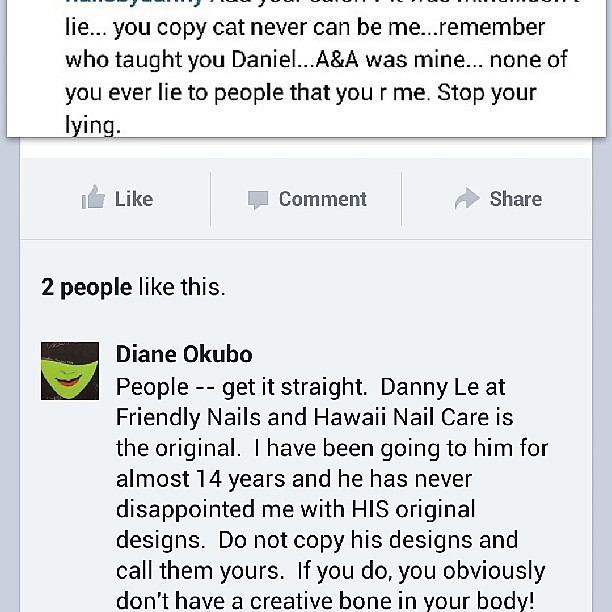The image is a screenshot from a Facebook post, showing a visibly cut-off top text that reads: "Lie... you copycat, never can be me... Remember, who taught you, Daniel? ANA was mine. None of you ever lie to people that you are me. Stop lying." The post has two likes and a comment from a user named Diana Akubo. Her profile icon depicts Elphaba, the green-faced witch from the show Wicked, characterized by a black hat shading her eyes and red lips shaped into a crooked smile. Diana's comment reads: "People, get it straight. Danny Lee at Friendly Nails and Hawaii Nail Care is the original. I have been going to him for almost 14 years and he has never disappointed me with his original designs. Do not copy his designs and call them yours. If you do, you obviously don't have a creative bone in your body." The screenshot is presented against a black and white background. The app interface, giving off visual cues typical of Facebook's design, takes up almost the entire frame.